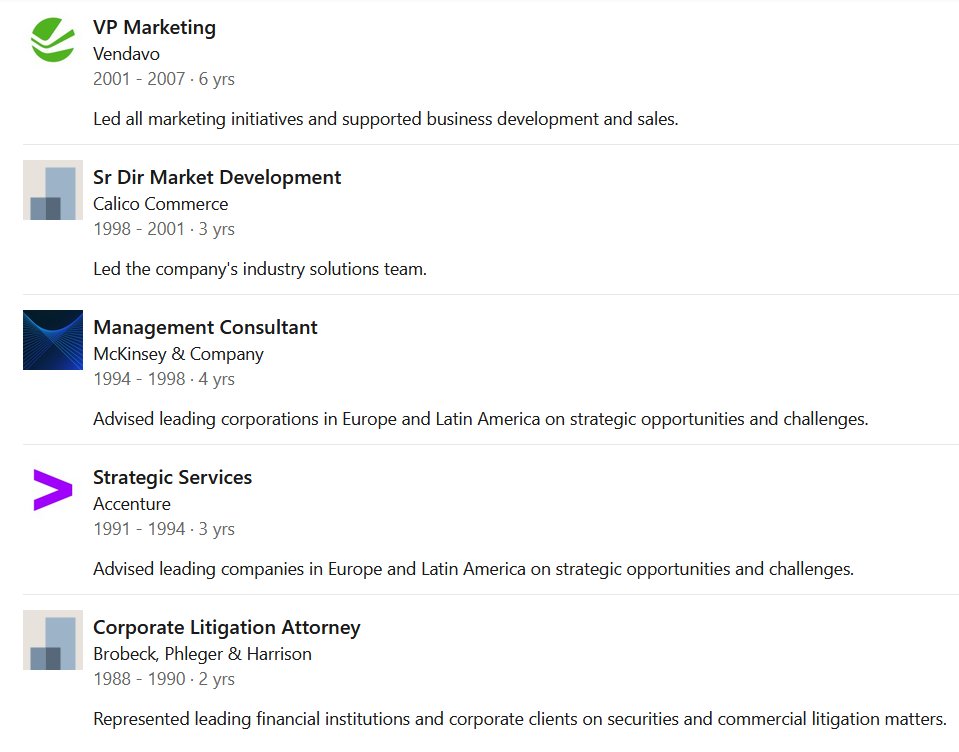A detailed professional timeline highlighting an extensive career in various high-level roles across multiple industries:

1. **VP of Marketing, Vendavo (2001-2007)**
   - Led all marketing initiatives.
   - Supported business development and sales activities.
   - Icon: Vendavo logo.

2. **Senior Director of Market Development, Calico Commerce (1998-2001)**
   - Led the company's industry solutions team.
   - Icon: Calico Commerce logo.

3. **Management Consultant, McKinsey & Company (1994-1998)**
   - Advised leading corporations in Europe and Latin America.
   - Focused on strategic opportunities and challenges.
   - Icon: McKinsey & Company textile logo.

4. **Strategic Services, Accenture (1991-1994)**
   - Provided strategic advice to leading companies in Europe and Latin America.
   - Concentrated on strategic opportunities and challenges.
   - Icon: Accenture purple arrow logo.

5. **Corporate Litigation Attorney, Brobeck, Flegger, and Harrison (1988-1990)**
   - Represented leading financial institutions and corporate clients in securities and commercial litigation matters.
   - Icon: Brobeck, Flegger, and Harrison standard gray rectangle logo.